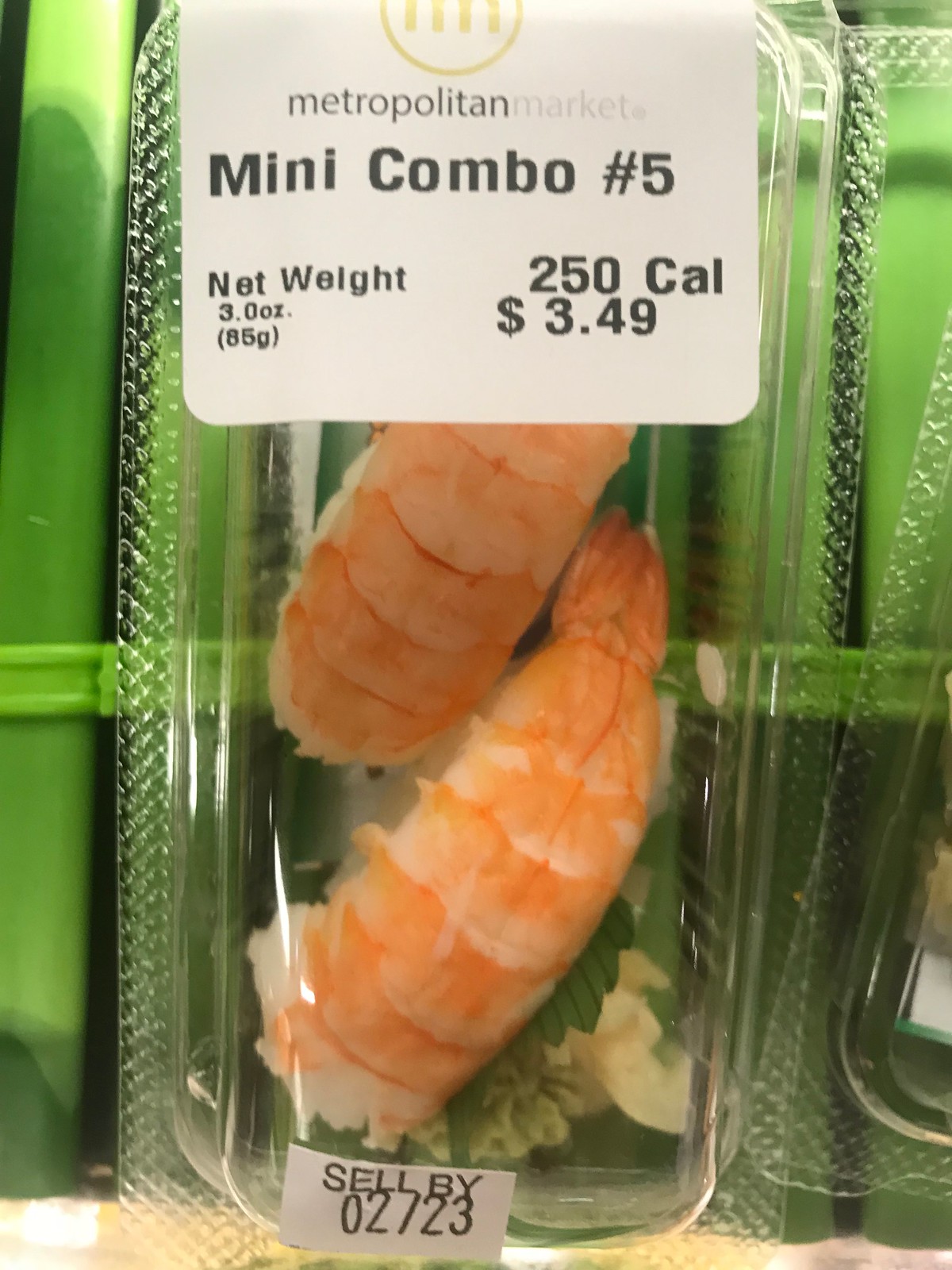This is a portrait-style image of packaged grocery store sushi taken inside a vending machine. The clear plastic container houses two pieces of sushi, each consisting of a white rice ball topped with a pinkish-orange shrimp tail. There is no nori paper, making them more like sashimi. The sushi sits on a green plastic leaf. The container has a top sticker that reads "Metropolitan Market, Mini Combo Number 5, net weight 3.0 ounces (85 grams), 250 calories, $3.49." A smaller sticker at the bottom indicates "Sell by 02-23." In the background, a green structure that resembles celery is partially visible. Another plastic container is seen to the right, cut off by the photo margins.